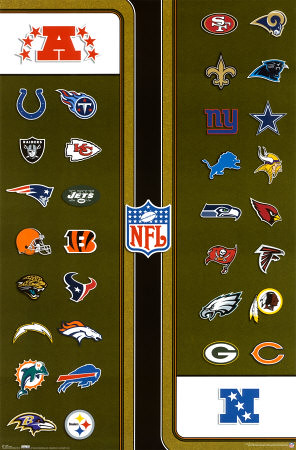The image displays a comprehensive collection of the 32 NFL team logos arranged by conference. The left side features the AFC teams, including the Miami Dolphins, Buffalo Bills, Cleveland Browns, Cincinnati Bengals, Las Vegas Raiders, Kansas City Chiefs, Baltimore Ravens, Tennessee Titans, Houston Oilers, New England Patriots, New York Jets, Carolina Panthers, Houston Texans, Los Angeles Chargers, Denver Broncos, and the Pittsburgh Steelers. The right side showcases the NFC teams like the San Francisco 49ers, Los Angeles Rams, New Orleans Saints, Carolina Panthers, New York Giants, Dallas Cowboys, Detroit Lions, Minnesota Vikings, Seattle Seahawks, Arizona Cardinals, Tampa Bay Buccaneers, Atlanta Falcons, Philadelphia Eagles, Washington Commanders, Green Bay Packers, and the Chicago Bears. Centrally positioned amidst these logos is the prominent NFL shield, unifying all the teams.